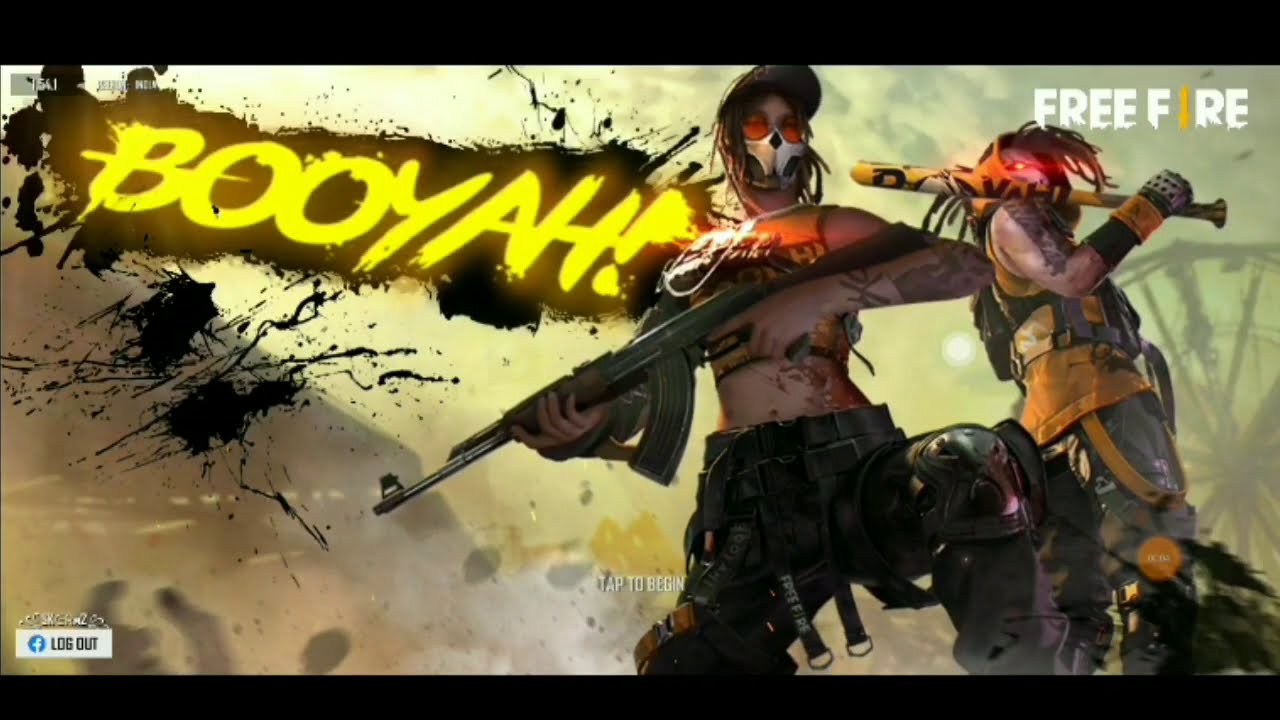This image is a vibrant and detailed screenshot from the menu screen of the game Free Fire, indicated by the white text with a yellow 'i' in the top right corner. The central focus of the image features an artistic dual portrait of two heavily armed characters in combat gear. 

On the left side, superimposed over a stylized background of black and brown paint splatters, the word "Booyah!" stands out in bright yellow, written in a bold and dynamic font. Below this resides social media options like logging out of Facebook.

The characters themselves are strikingly detailed. The character in the foreground, who appears female, faces the viewer. She wears utility cargo pants and a yellow crop top, accessorized with a white mask covering her lower face, red sunglasses, and a ball cap. Her arms are tattooed, and she holds an AK-47 across her body in a poised, ready stance.

To her right is another character, whose back is partially turned towards the viewer. This character, with long flowing hair and glowing red eyes, rests a black-and-yellow baseball bat on their shoulder. They are similarly outfitted with combat gear including chest and waist gear, knee pads, and gloves.

The entirety of this evocative scene is set against a muted, blurred background of yellowish and brownish hues, offering a sharp contrast to the clear and vibrant details of the characters in the foreground.